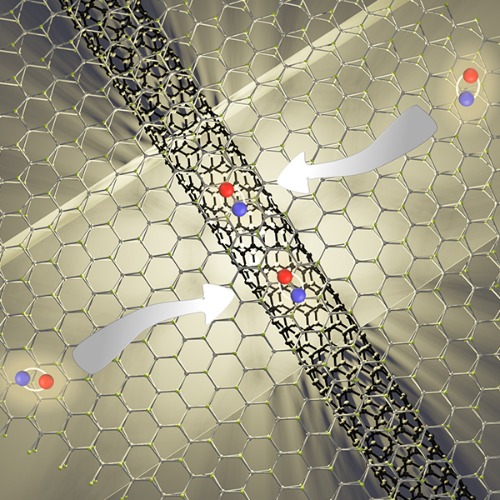The image depicts a detailed computer-generated visual representation of carbon nanotubes. The background features a hexagonal grid that resembles a wire mesh or chicken wire, with the hexagons predominantly silver, except for a central tube where the hexagons are black. This black hexagonal tube runs diagonally from the upper left to the bottom right of the image. Two prominent white curvy arrows, originating from opposite corners of the image, point towards the central tube, each terminating at a point where a red and blue sphere is connected. Surrounding this central structure are additional red and blue spheres, each pair connected by ellipsis-shaped silver rings. The background is illuminated by a glowing white rectangle that resembles a plastic light fixture, casting a radiant glow that highlights the entire setup. This intricate model appears to depict the interaction and arrangement of molecular structures within carbon nanotubes, with yellow dots marking the corners of the hexagonal grid and white tubes forming the hexagonal lines. The overall appearance is both scientific and artistic, capturing the complexity of nanomaterial arrangements.